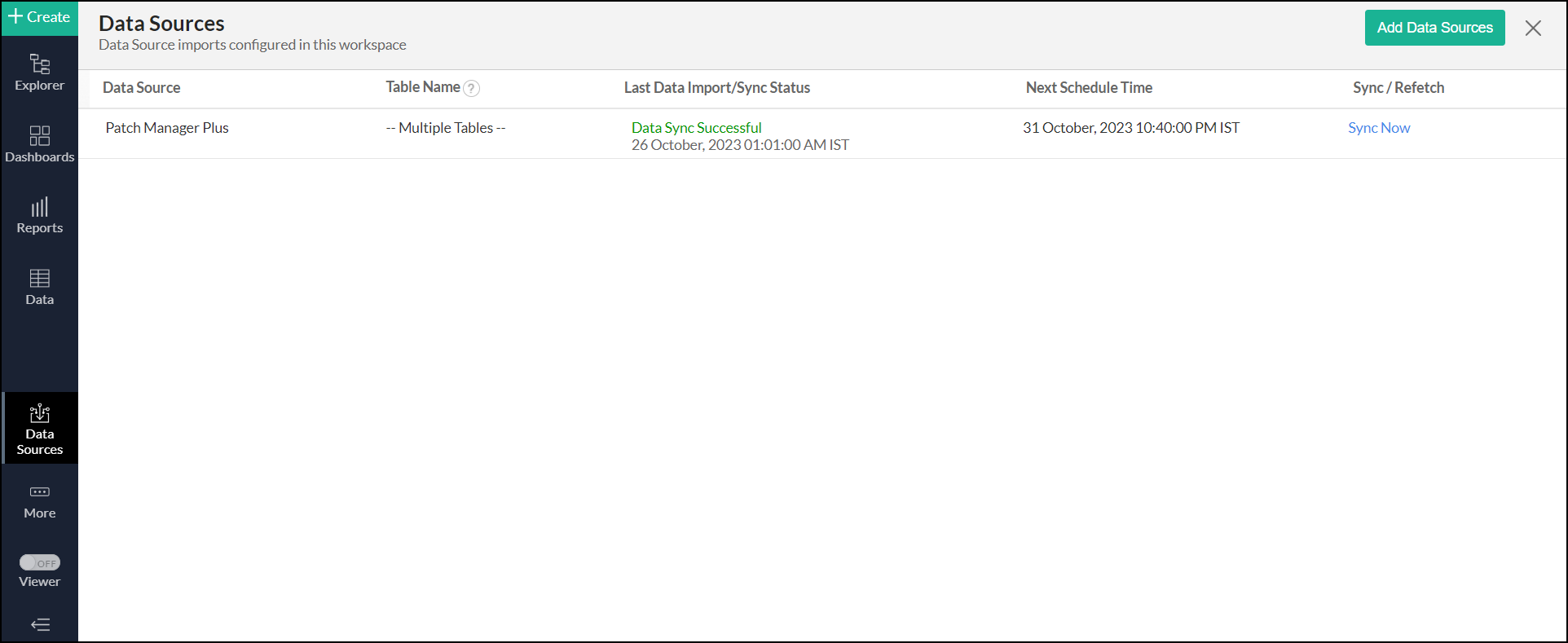The image is a screenshot from a website interface that displays various data source configurations. At the top of the image, there's a heading that reads "Data Sources". Directly below this heading, in smaller print, is the description "Data source imports configured in this workspace".

Beneath this, there is a column labeled "Data Source", under which "Patch Manager Plus" is listed. Adjacent to this, there's another column labeled "Table Name" which states "Multiple Tables". 

Further down, a section labeled "Last Data Import/Sync Status" indicates that the "Data Sync" was successful, with the timestamp "26 October 2023". Additionally, the next scheduled time for the data import/sync is shown as "31 October 2023, 10:40 PM IST". 

The last column is labeled "Sync/Refresh" and includes a button in blue text labeled "Sync Now", which can be clicked to synchronize the data immediately.

At the very top right of the screen, there's a green button labeled "Add Data Sources".

On the far left-hand side of the screen, there is a vertical navigation bar with the following options, each accompanied by an icon: "Explorer", "Dashboards", "Reports", "Data Search", "Data Sources", and "More". Below these, there's an option labeled "Viewer".